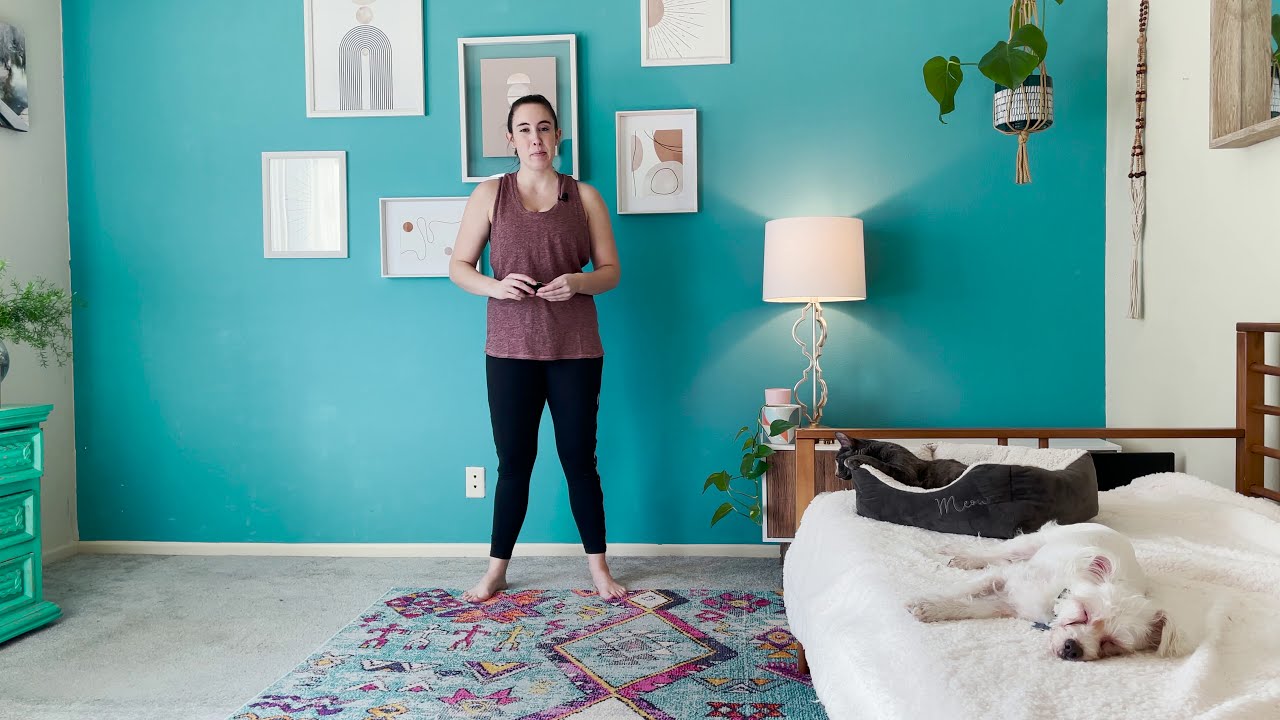In this photograph, a Caucasian woman in her 20s is standing barefoot in her bedroom, slightly left of center. She is wearing tight black leggings and a dark maroon sleeveless tank top. Her brown hair is neatly pulled back. She is looking directly at the camera with her hands almost together in front of her. The room features a teal wall behind her adorned with various framed photographs and possibly certificates. The adjacent walls are white, creating a contrasting backdrop.

To her right is a daybed or futon covered in white bedding, upon which a white dog is peacefully sleeping. Behind this dog is a gray dog bed. Additionally, a black or dark brown cat bed with embroidery reading "meow" is present but not immediately noticeable. The lower right corner of the image includes another lamp, which is turned on, sitting on a wooden desk or cabinet. There's a plant hanging in the upper right corner of the room, adding a touch of greenery.

The floor is gray tile, overlaid with a multicolored rug featuring patterns of light greens and red triangles, as well as varying designs in blue, purple, and pink hues. The atmosphere appears cozy and personalized, with the various elements and décor hinting at a lived-in, comfortable space.